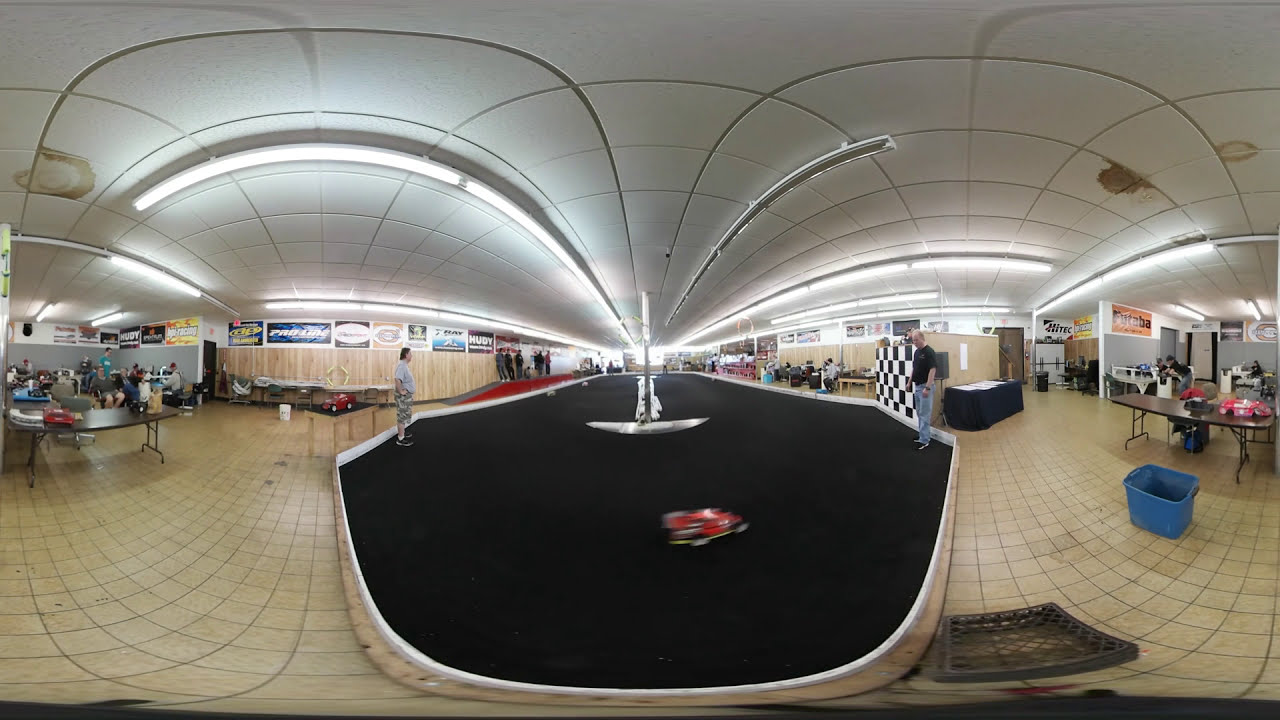The image showcases a bustling, large convention center with a distinct, scalloped white domed ceiling adorned with a grid of powerful, evenly distributed lights. Taken with a fisheye lens, the picture exhibits a slight distortion that captures the grandeur of the room in its entirety. At the center, an elevated, pitch-black stage surrounded by a white border stands out, featuring two men possibly setting up for an event. To the right of this stage, we notice a checkered black-and-white wall which seems to demarcate an indoor racetrack for radio-controlled cars, with a blurry red car in motion and another stationary car on a nearby folding table. The room is filled with glass tables and chairs, populated with attendees who blend into the background. Sponsorship logos and placards embellish the walls, hinting at an auto-themed event, further suggested by a red symbol on the stage. The long, large building buzzes with preparations and hints of competitive excitement, making it a dynamic, multifaceted scene.